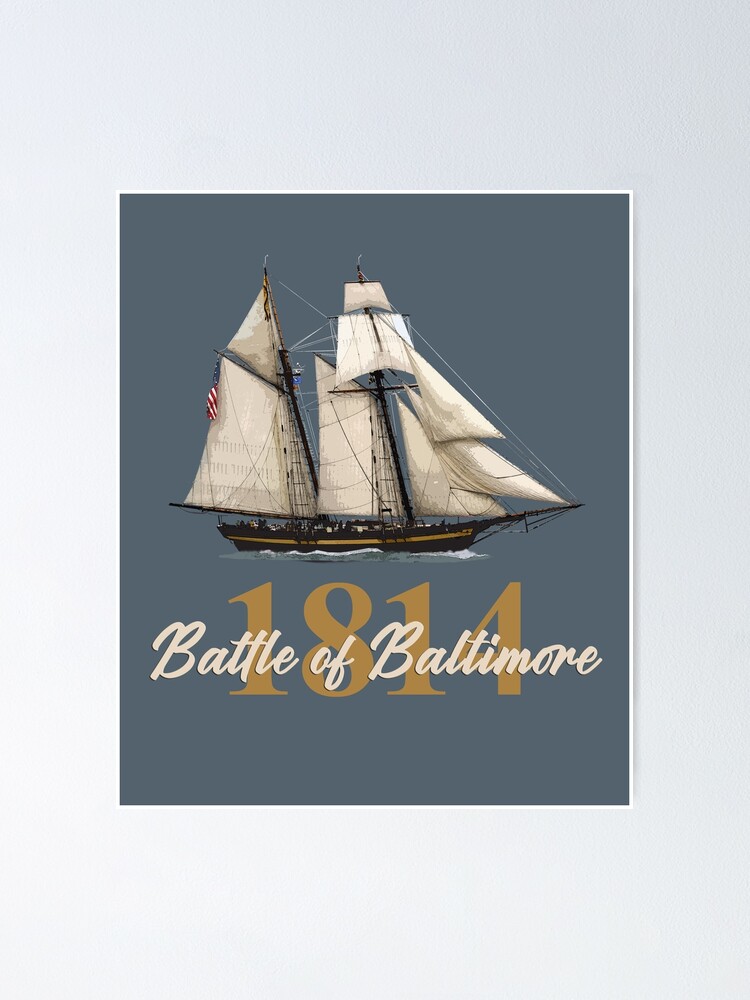A vibrant image set against a blue binder background, bordered by a gray frame, showcases a historically themed illustration. At the center, prominently displayed in large gold numbers, is "1814," marking the year of the significant event depicted. Above these numbers, there is a meticulously detailed illustration of a brown ship adorned with a gold stripe running along its hull. The ship is equipped with two white sails mounted on sturdy masts and features a long bowsprit extending from the front. Additionally, an American flag flutters at the stern, connected by an array of rigging ropes. Below the ship, the text "Battle of Baltimore" is presented in bold white letters, further emphasizing the historical context of the image.